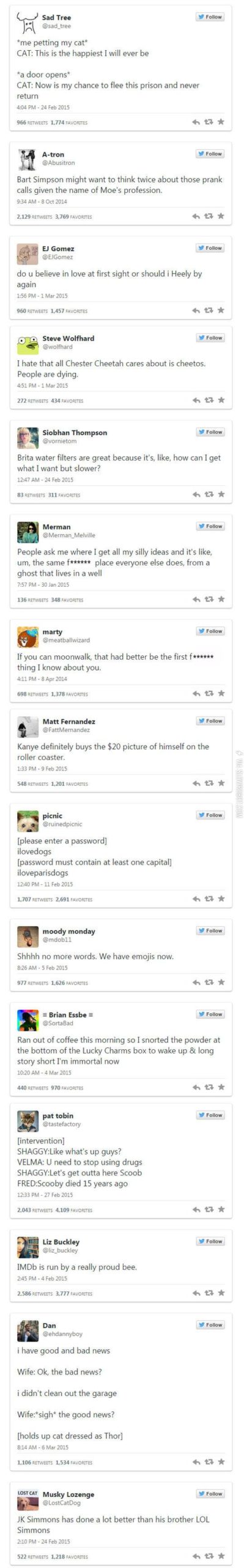The cropped, low-resolution image features a primarily white background showcasing a vertical list of horizontally-aligned sections. Each section includes a small, unclear picture in the upper left corner, potentially depicting cars or assorted items, though they are mostly indistinct blotches. Adjacent to the images, there are brief blocks of text, typically consisting of two to three sentences. Below the text in each section, there are three unreadable buttons. Some blue links might be present, but the resolution is too low to confirm. Each section seemingly has a header, likely indicating the name of a vehicle, object, service, or goods. On the far right side of the image, there's a faint, vertically oriented, off-white rectangle, presumably a scroll bar.